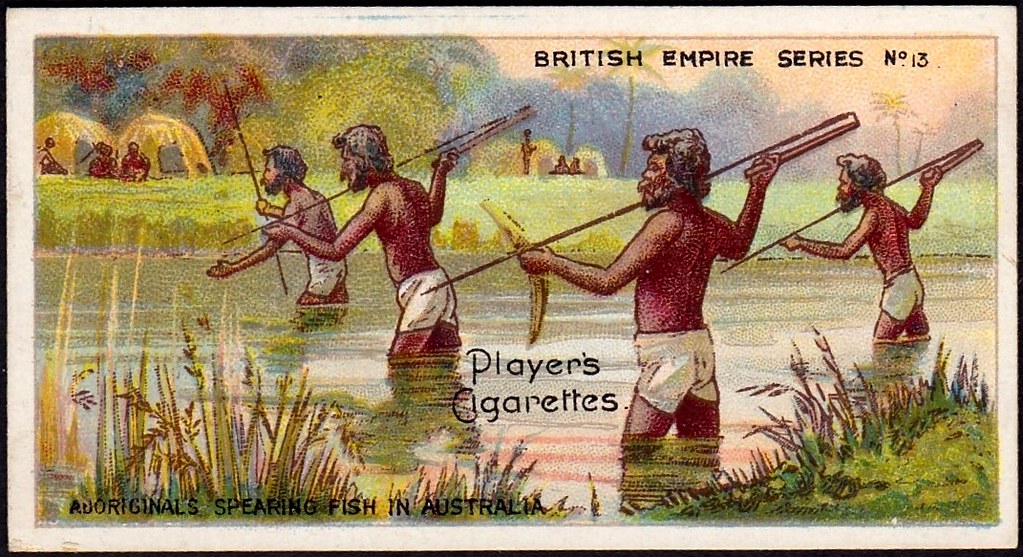The image is a vintage, colorful advertisement with a cartoonish feel, featuring a scene of Aboriginal men engaged in spearfishing in Australia. The setting depicts a river running horizontally across the middle of the image, surrounded by lush greenery and tall reeds. The men, depicted with dark skin, are knee-deep in the vibrant blue water, wearing white swimming trunks, and holding spears. They are all focused on their fishing, with one man positioned prominently at the front, his spear raised beside his shoulder. The background shows a grassy area dotted with several brown huts and people sitting in front, amidst green and brown trees.

The advertisement prominently showcases the text "Players, Cigarettes" in the middle of the water, indicating the promotion of the cigarette brand. At the top right, the text "British Empire Series No. 13" is written in black, while the bottom left corner features the caption "Aboriginals Spearing Fish in Australia." The entire illustration is framed with a cream-colored mat and a black border, enhancing its classic, vintage allure.